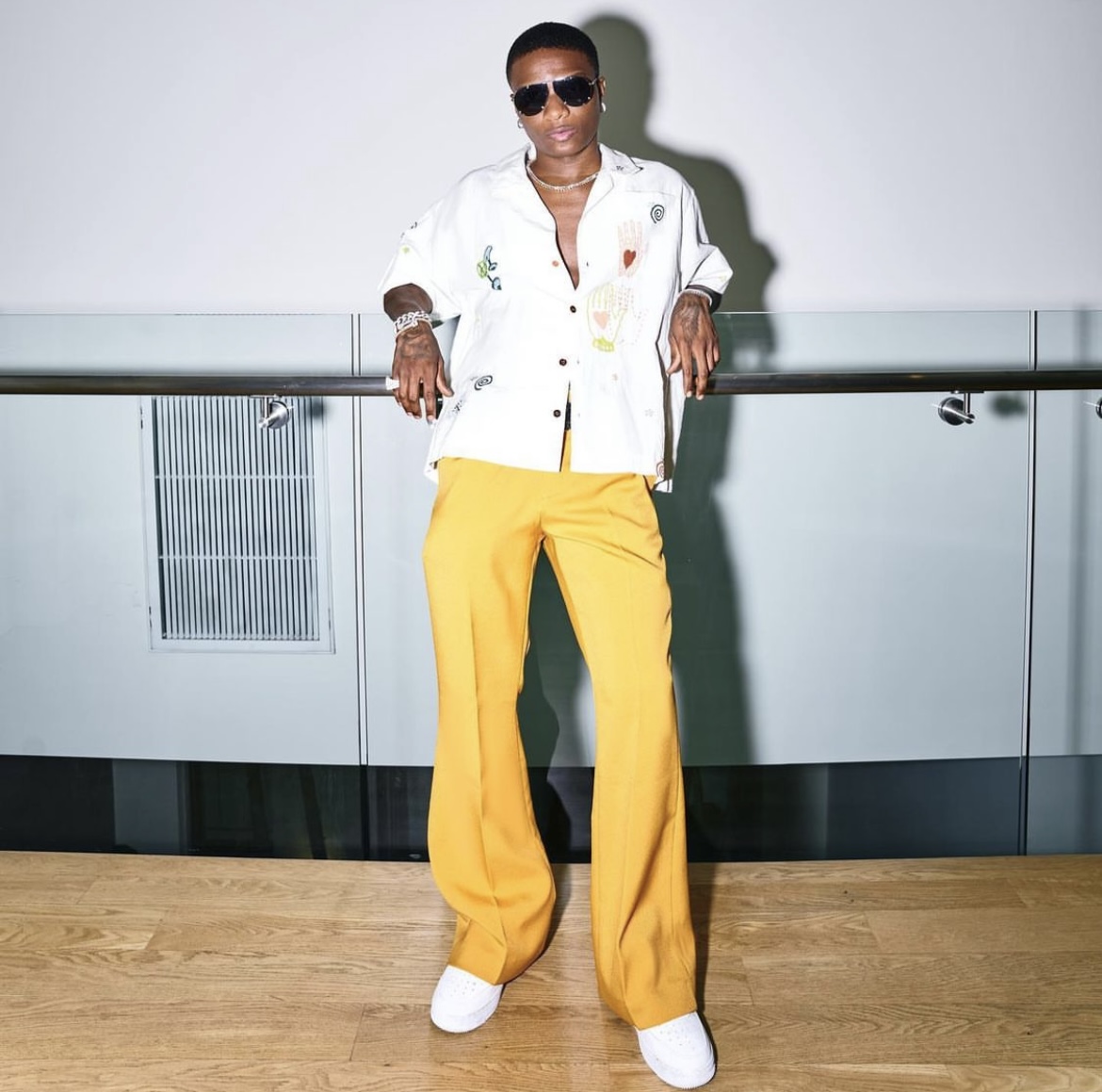The image depicts an African-American man with dark brown skin and very short hair, leaning against a dark brown railing in front of a clear glass wall. He is wearing yellow pants and a matching cream-colored shirt adorned with embroidered hearts, one of which is the same color as his pants. The man has white tennis shoes on his feet and is accessorized with dark sunglasses, earrings, a necklace, rings, bracelets, and a watch. The floor beneath him is light brown wood. Given his relaxed yet confident demeanor and the stylish outfit, he could be in a leisure setting like a cruise ship, an entertainment venue, or another public space.